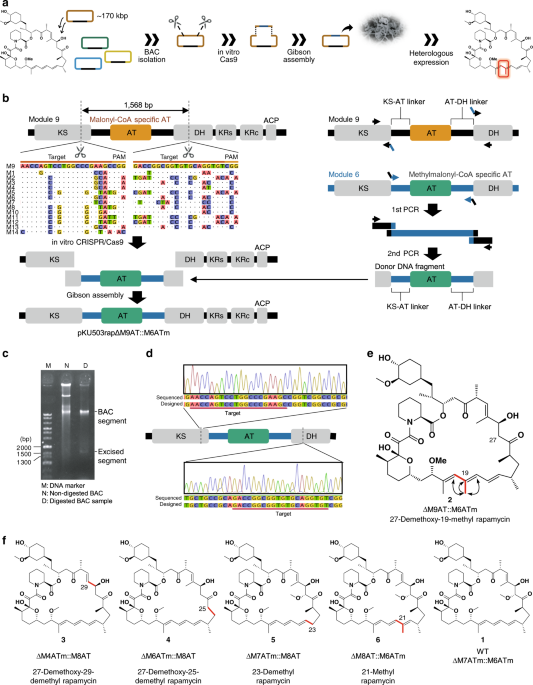The image appears to be an intricate page from a textbook or an educational manual, featuring numerous, highly detailed diagrams related to chemical compounds and molecular structures. Each diagram is meticulously labeled, with sections denoted as A, B, C, D, E, and F columns, among others, indicating the various parts and their interconnections. The illustrations include both colored and black-and-white elements, with arrows linking different modules and numerous scientific annotations. The complexity and absence of an overarching title make it challenging for those unfamiliar with the subject to discern the exact nature of the content, suggesting it requires specialized knowledge to fully understand.